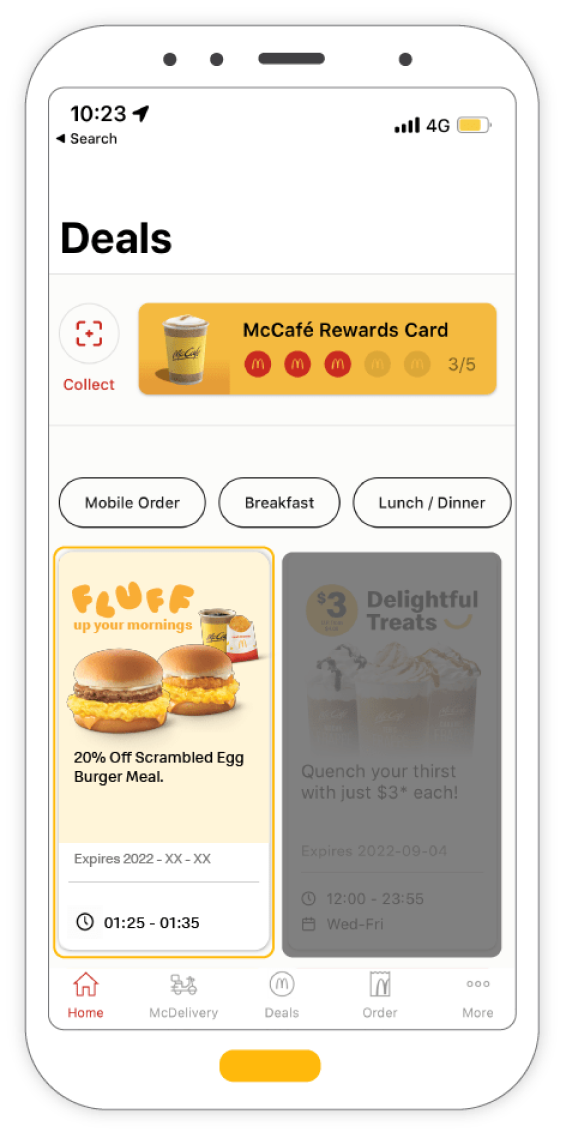This image showcases an artistic rendering of a smartphone displaying the McDonald's mobile app interface. The drawing features a white phone with two dots on the top left, presumably sensors or cameras, and a speaker grill on the top right.

At the top left of the screen, the time reads 10:23, while the top right shows a full cell signal (four out of four bars), 4G connectivity, and a battery level at 83%. Below these icons, the primary navigation includes a black "Deals" tab, a prompt to "Tap to Collect," and the McCafé Rewards card with three out of five McDonald's symbols filled.

Scrolling down, the interface offers tabs labeled "Mobile Order," "Breakfast," "Lunch," and "Dinner." Promotional content includes an offer for "20% off Scrambled Egg Burger Meal," valid until 2022 with no specific expiration date mentioned. Another offer highlights "Delightful Treats" available for $3, emphasizing affordability with the statement "Quench your thirst with just $3 each."

At the bottom of the screen, additional navigation tabs can be seen for "Home," "McDelivery," "McDeals," "Order," and "More."